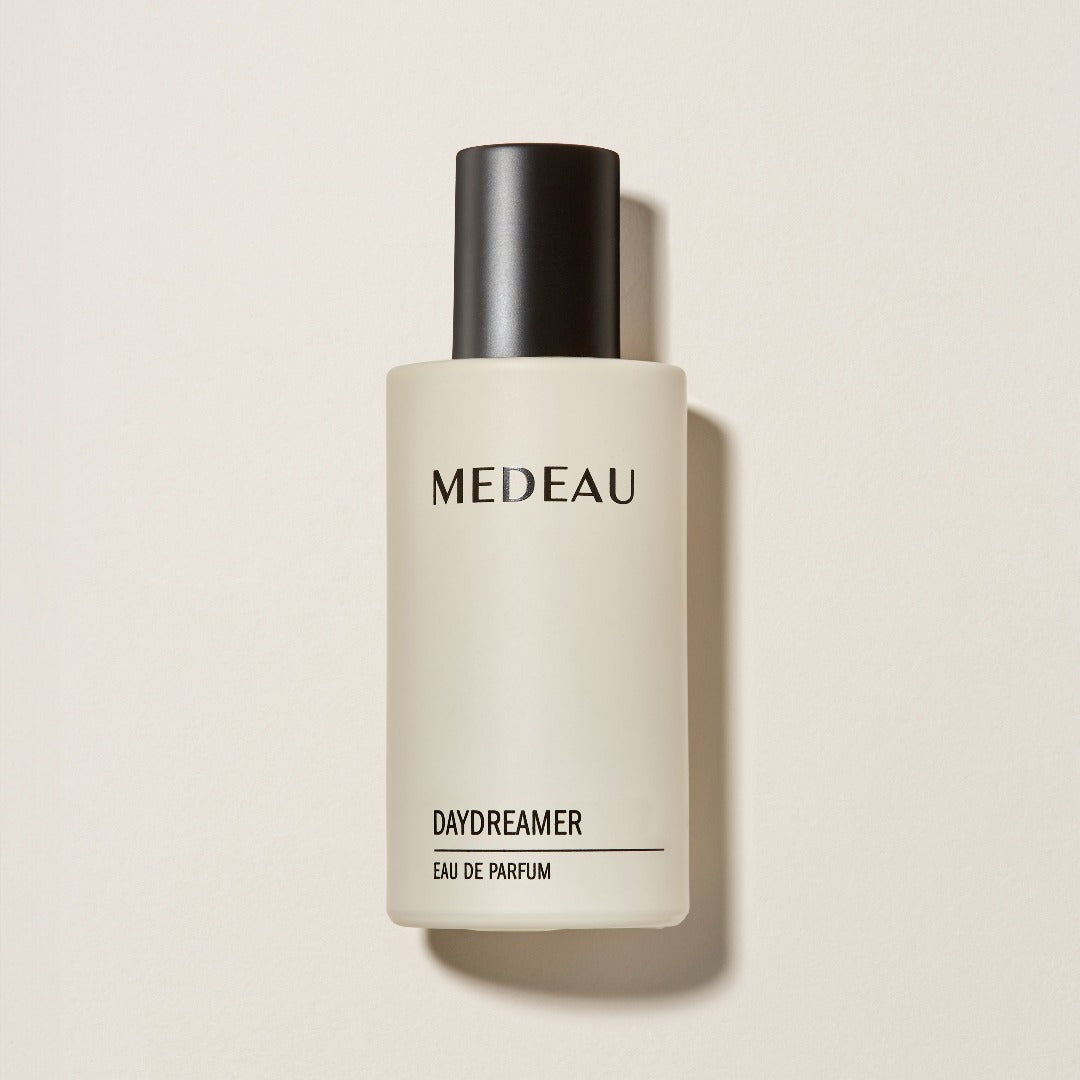The image is a square, six inches wide and six inches tall, featuring a plain off-white background without any additional borders. At the center of the image, there is a bottle of perfume measuring approximately one inch wide by three inches high. The bottle is made of frosted glass that blends seamlessly with the off-white background. It has a cylindrical black cap, which is about half an inch to three-quarters of an inch wide and one inch tall. The design on the bottle is minimalist, featuring the brand name "MEDEAU" written in all caps at the top portion, in black sans serif font. Lower on the bottle, also in black all caps, is the word "DAYDREAMER," followed by a thin horizontal line. Beneath this line, the text "EAU DE PARFUM" is displayed. The bottle casts a subtle shadow to the right and bottom, adding depth, which makes the bottle appear elliptical when viewed from the top or bottom. The overall composition creates a visually clean and focused representation of the product, making it unclear if the image is a hyper-realistic drawing or a photograph.